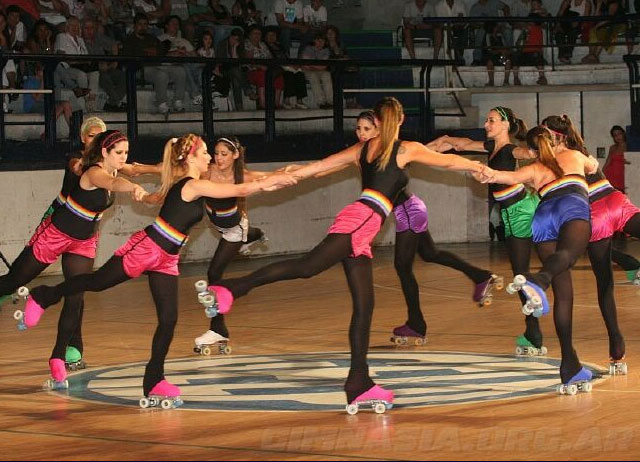The color photograph, captured indoors, depicts a lively scene of a group of women roller skating in a circle on a wooden stadium floor, possibly reminiscent of an earlier era. The skaters are all dressed in coordinated outfits featuring black tops and black stockings, with a distinctive multi-colored belt—red, yellow, and purple—around their waists. Their shorts and roller skates share matching vibrant hues: pink, blue, green, purple, and white. Each skater's wheels on their roller skates are also color-coordinated. The women are holding hands while performing a symmetrical skating routine, which suggests a choreographed performance.

An audience is visible in the background, seated in grandstands with a black railing, seemingly made of stone or cement, attentively watching the spectacle—potentially a main show or halftime event. Additionally, the image details a watermark, difficult to read, indicating a website ending in ".org.ar". Other individuals, possibly skaters preparing for their routine, can be seen in a designated area to the left of the rink, adding to the dynamic atmosphere of the scene.